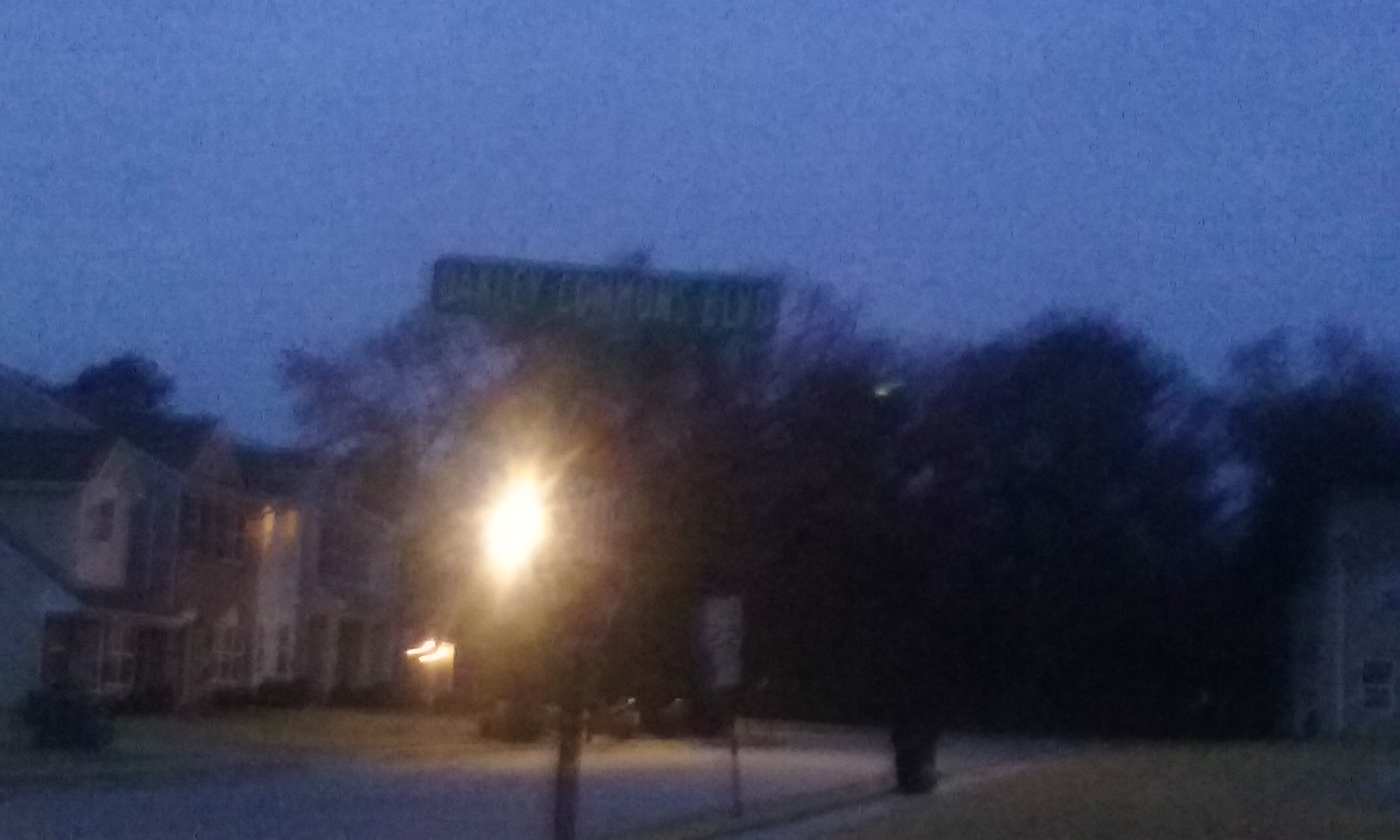This blurry photograph captures a suburban neighborhood at dusk, with the sky darkening to a deep blue. The scene is illuminated by several streetlights, one of which casts a starburst halo. In the foreground, partially obscured by a nearby streetlight, stands a red and white octagonal stop sign, above which is a green street sign with white lettering that reads "Oakley Commons Blvd." A white speed limit sign, though blurry, appears beside the stop sign.

The street runs diagonally from the bottom left corner of the image towards the center, where it seems to dead-end into a dense cluster of trees. On the left side of the photograph, four houses line the street, each with some exterior lights on. The houses include a white one, a seemingly dark brown one, another white and gray one, and a partially obscured house revealing limited details due to the poor lighting. On the right-hand side of the image, there's a partial view of another house. Additionally, a couple of parked cars can be spotted along the street, blending into the grainy, dimly lit scene.